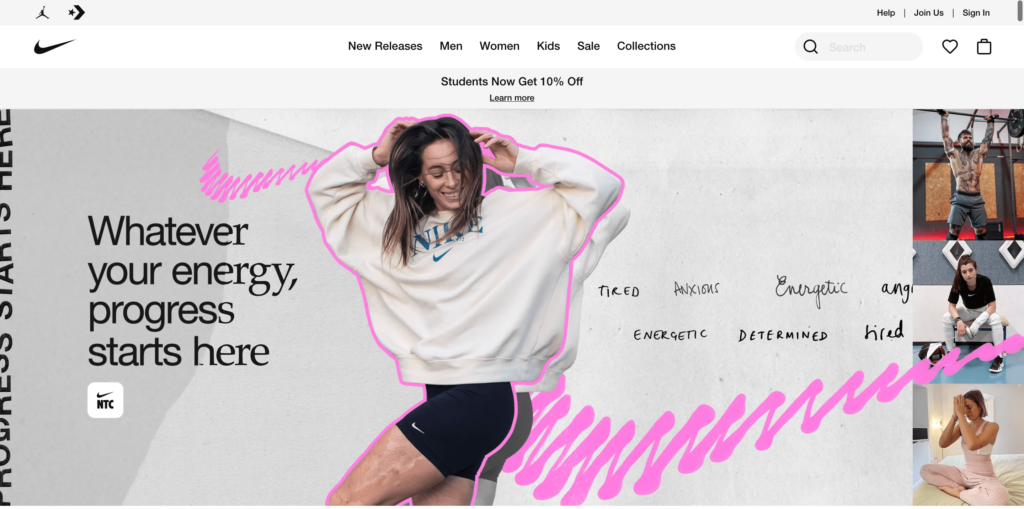This rectangular image, oriented horizontally, appears to be promoting a fitness app or website, likely affiliated with Nike. At the top, a light gray banner spans the width of the image. On the left side of this banner, the iconic Michael Jordan "Jumpman" logo, along with the Nike "swoosh" symbol, is displayed, suggesting that this is indeed a Nike page. Adjacent to these symbols are a star icon and a right-pointing arrow. On the far-right of the banner, the text options for "Help," "Join Us," and "Sign In" are clearly visible.

Below this, a white navigation bar extends across the top. On the far left of this bar is the black Nike "swoosh" symbol. Centrally, the navigation options show "New Releases," "Men," "Women," "Kids," "Sale," and "Collections." Towards the right, there is a gray circular search icon featuring a black magnifying glass, a heart symbol, and what appears to be a shopping cart icon.

Further down, another light gray banner announces, "Students now get 10% off, learn more."

Finally, the main body of the website is revealed. On the far left, vertical text partially extends out of the frame, and next to it, in bold letters, the motivational phrase reads, "Whatever your energy, progress starts here." This welcoming message sets the tone for users to begin their fitness journey with Nike.